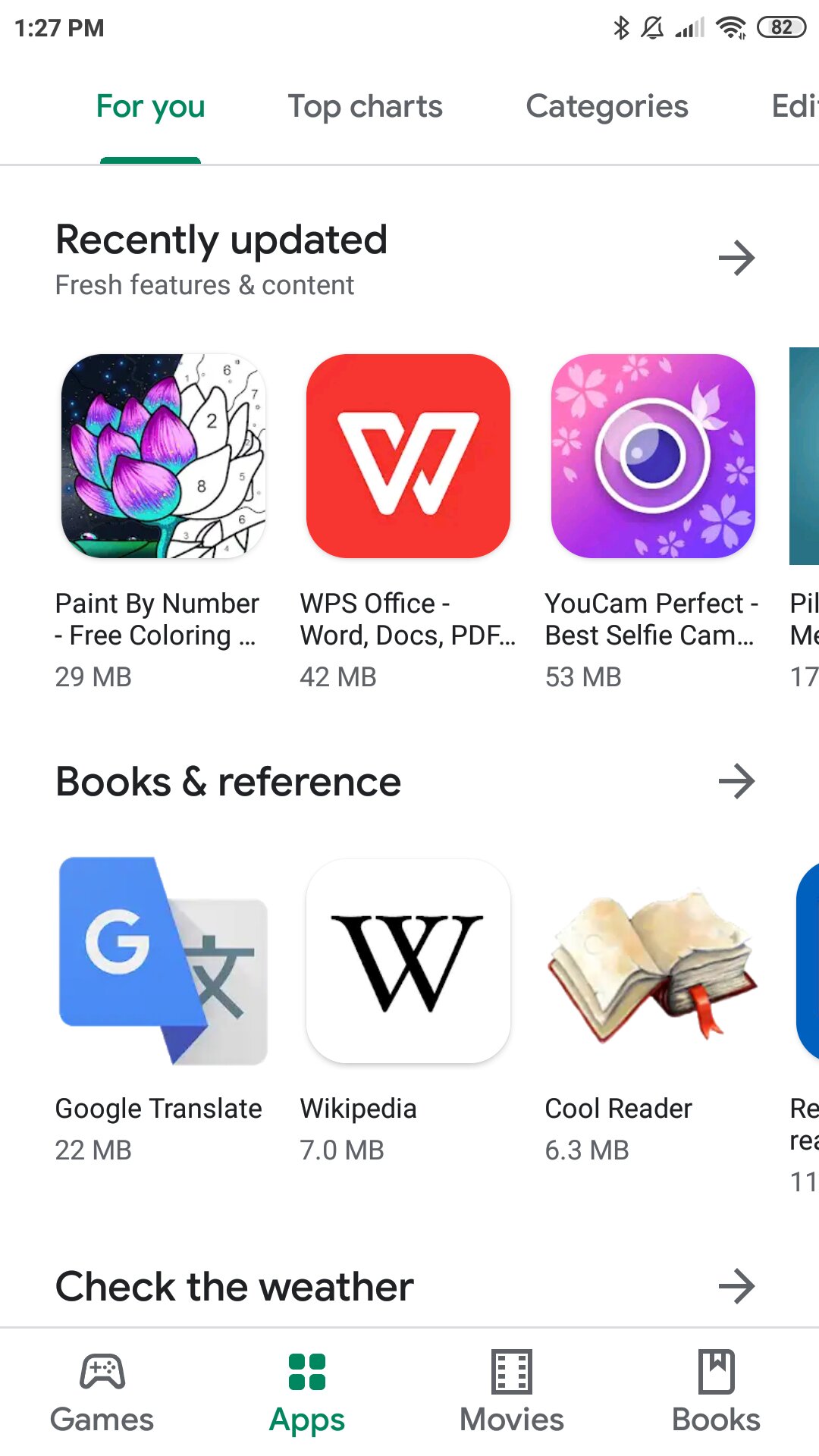This detailed screenshot displays a section of a mobile app store interface, focusing on various apps available for download. At the top of the screen, there are navigational tabs: "For You" highlighted in green, followed by "Top Charts," "Categories," and "Edit," all in gray. Below these tabs, the heading "Recently Updated" is in black, with the subheading "Fresh features and content" in smaller gray font.

The first app listed is "Paint by Number - Free Coloring," occupying 29 MB of space. The app icon features an image of a partially colored, vibrant purple and green flower on a black background, juxtaposed against a numbered, uncolored section. 

Next, there is the "WPS Office - Word Docs PDF" app, which takes up 42 MB. Its icon is a red square with a creatively designed white "W."

Following this is the "Ucam Perfect - Selfie Cam," identified by its 28 MB size. The icon is a gradient square shifting from pink at the top to purple at the bottom, featuring a camera lens and floral decorations.

A new category labeled "Books & Reference" begins on the next row. Here, "Google Translate," consuming 22 MB, is represented with an icon split between a "G" on one side and a gray foreign language character on the other.

Next to it is the  "Wikipedia" app, sized at 7.0 MB, with a simple white square and a "W" on it.

Following this is the "Cool Reader" app, at 6.3 MB, depicted with an open book icon showcasing yellowed pages and a red bookmark.

Further down, a prompt reads "Check the weather" in black text.

At the bottom of the screen are the navigation icons for Games, Apps, Movies, and Books. All are in black except for "Apps," which stands out in green.

This detailed description captures the layout and specifics of the interface, providing a comprehensive look at the various apps and their icons.